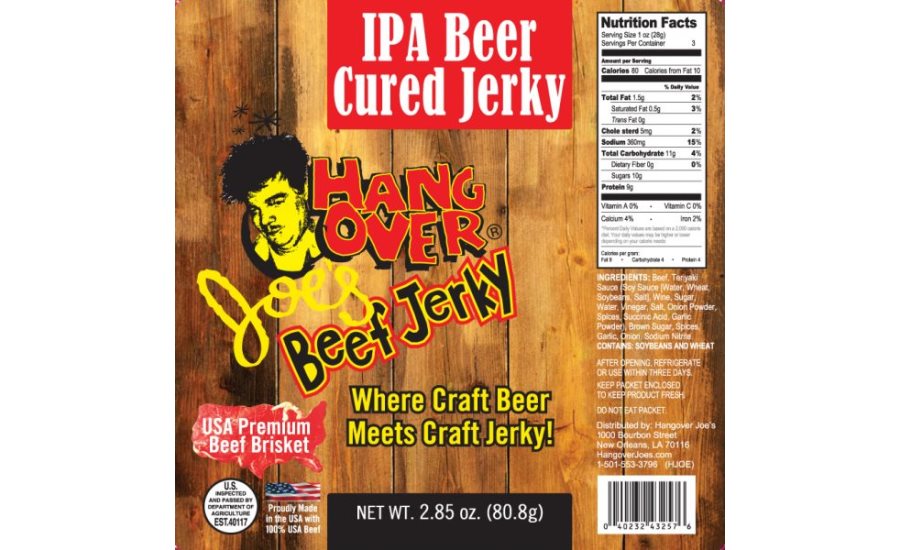This image depicts a detailed label for Hangover Joe's Beef Jerky, highlighting its IPA Beer Cured Jerky. The label features a wooden fence background that exudes a rustic charm. Prominently displayed at the top center in a red rectangle with white capital letters is "IPA Beer," followed by "Cured Jerky." The lower left section in red letters reads "Hangover," with "Joe's" in cursive yellow lettering below it. "Beef Jerky" is written underneath in black font, and the slogan "Where Craft Beer Meets Craft Jerky" follows in yellow letters with a black outline.

The label emphasizes the jerky's high-quality ingredients, noting it is made from USA premium beef brisket. An image of a man who appears as though he might be hungover, with chaotic, spiky black hair and a yellow face, is featured next to the word "Hangover." The net weight of the package is specified as 2.85 ounces (80.8 grams).

Nutritional information is detailed on the right side in a traditional black and white format, noting that a serving size is 25 grams, which contains 80 calories, 1.5 grams of fat, 5 milligrams of cholesterol, 360 milligrams of sodium (15% of daily value), 11 grams of total carbohydrates (4% of daily value), and 9 grams of protein. It also contains 2% iron and 4% calcium per serving. There are approximately three servings per box or container.

Additional elements on the label include a barcode at the bottom right, a USA inspection tag at the lower left, and instructions indicating that the jerky should be refrigerated or consumed within three days after opening.